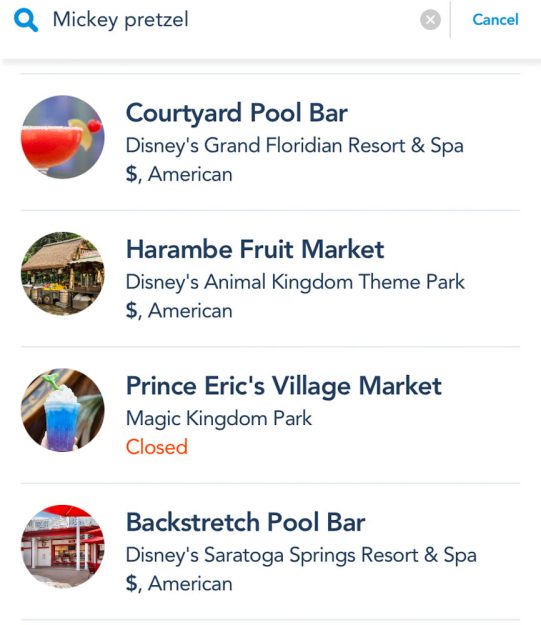This is a detailed screenshot likely from a travel app or website featuring dining options. At the top, a search bar reads "Mickey Pretzel" with a "Cancel" button and an adjacent "X" icon. Below, a list of venues appears:

1. **Courtyard Pool Bar, Disney's Grand Floridian Resort and Spa** - An image of a fruity drink accompanies this venue, listed under the category "American" with a single dollar sign ($), indicating affordability.
2. **Harambee Fruit Market, Disney's Animal Kingdom Theme Park** - Depicted with an icon of a small hut-like structure, this venue is also categorized as "American" and marked with a single dollar sign ($).
3. **Prince Eric's Village Market, Magic Kingdom Park** - Features a colorful icy drink in white, blue, and purple. This venue is currently listed as closed.
4. **Backstretch Pool Bar, Disney's Saratoga Springs Resort and Spa** - Shown with an icon of an exterior restaurant venue, categorized under "American" with a single dollar sign ($).

The layout suggests this is from a mobile app, given its compact, scrollable design suited for smaller screens. The background is white, enhancing clarity and readability.